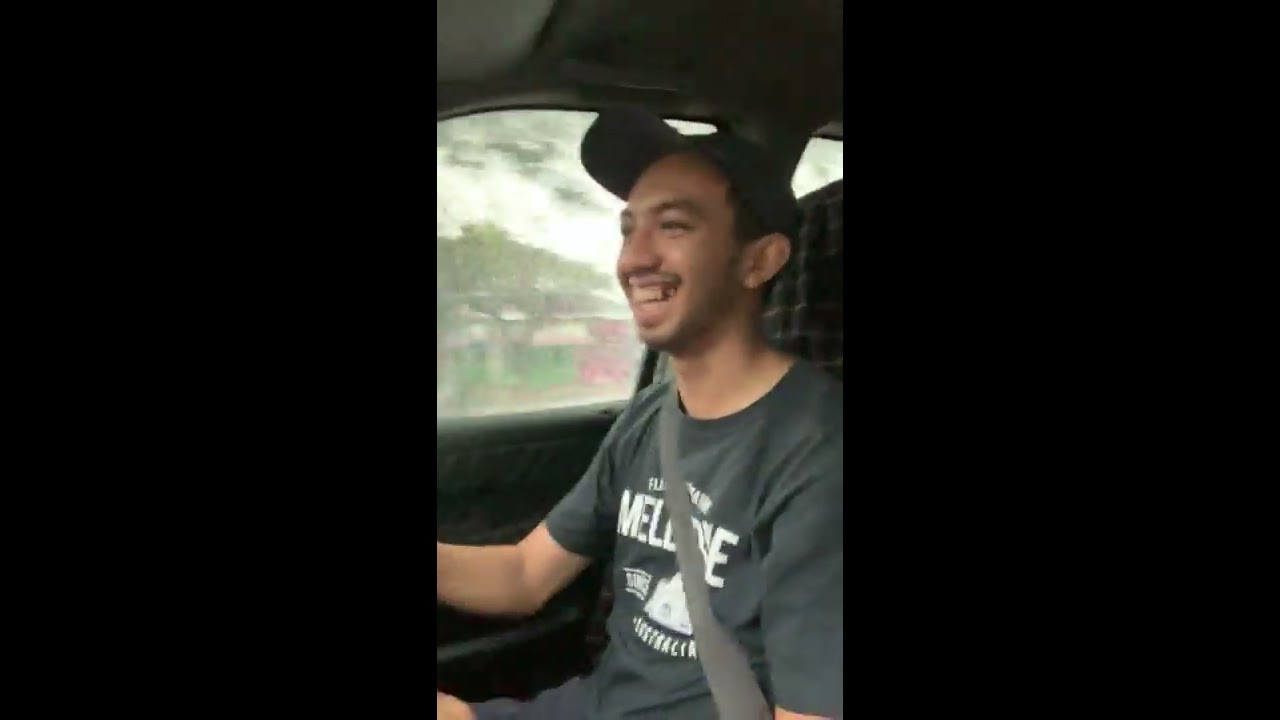The image features a slender young man in his early 20s, seated in the passenger seat of a moving car. He has a warm, cheerful smile on his face, revealing a gap in his teeth on the left side. The man is of Middle Eastern descent, with brown skin and a slight mustache and five o'clock shadow. He wears a black baseball cap and a gray short-sleeved t-shirt with a white graphic design that might read "Melbourne." His seatbelt is fastened securely across his chest. Behind him, the checkered pattern of the headrest is visible, and outside the window, the blurry outdoor environment indicates that the car is in motion. The photograph, taken in vertical cell phone format, has been placed into a landscape frame, resulting in black bars on the left and right sides. The overall lighting suggests an overcast day, with no direct sunlight.